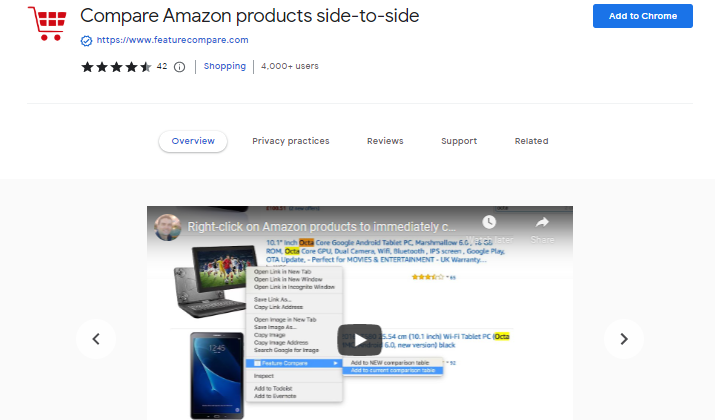This screenshot showcases a browser extension available for Chrome, designed to enhance the shopping experience on Amazon. The primary feature, emphasized by a prominent blue "Add to Chrome" button, is the ability to compare Amazon products side by side easily. Highlighted within the interface are various elements such as an overview tab, a red shopping cart icon, and a concise description of the extension's core function: enabling users to compare Amazon products seamlessly.

The extension boasts 42 positive reviews and over 4,000 users, indicating its popularity and reliability. It falls under the 'Shopping' category, with a specific focus on feature comparison shopping. Additional tabs available include privacy policies, reviews, and support, providing comprehensive information and user assistance.

The page also features an embedded video, which users can play to gain a detailed understanding of the extension's functionalities. The video thumbnail displays icons of different devices—including a computer, laptop, phone, and tablet—implying multi-device compatibility. Notably, a highlighted instruction on the thumbnail advises users to right-click on Amazon products to quickly compare them, with arrows indicating forward and backward navigation options.

Below, the user reviews, support options, and related extensions are accessible, offering further insights and assistance to potential users. This thorough layout ensures that all necessary information about the extension is readily available, making it user-friendly and informative.